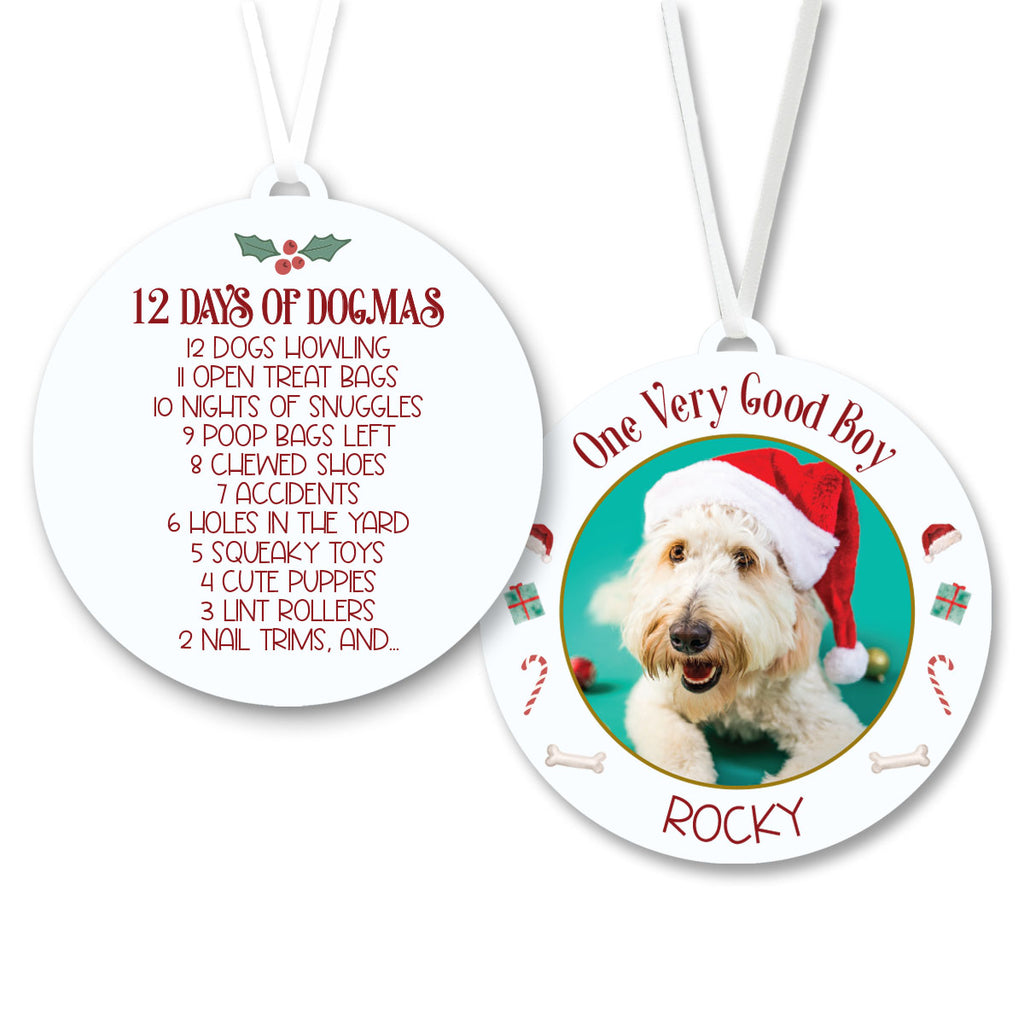This detailed image depicts two flat, circular Christmas ornaments, each with a notch at the top threaded with a white satin ribbon, presenting both the front and back views. The left ornament showcases a festive design with holly and red berries at the top, against a clean white background. In dark red, Christmas-themed lettering, it reads "12 Days of Dogmas" at the top, followed by a whimsical list: "12 Dogs Howling, 11 Open Treat Bags, 10 Nights of Snuggles, 9 Poop Bags Left, 8 Chewed Shoes, 7 Accidents, 6 Holes in the Yard, 5 Squeaky Toys, 4 Cute Puppies, 3 Lint Rollers, 2 Nail Trims, and ...".

The opposite side features a similar circular ornament with an arched red inscription, "One Very Good Boy." Inside an inner blue circle, a cute white schnauzer wearing a Santa hat rests with its paws outstretched. Below the delightful portrait is the name "Rocky" in bold red letters. Surrounding the inner circle are festive icons, including candy canes, presents, Santa hats, and bones, which enhance the holiday spirit of the design. This realistic, photographic representation combines graphic design elements, making these ornaments both a charming holiday decoration and a personalized celebration of a beloved pet.